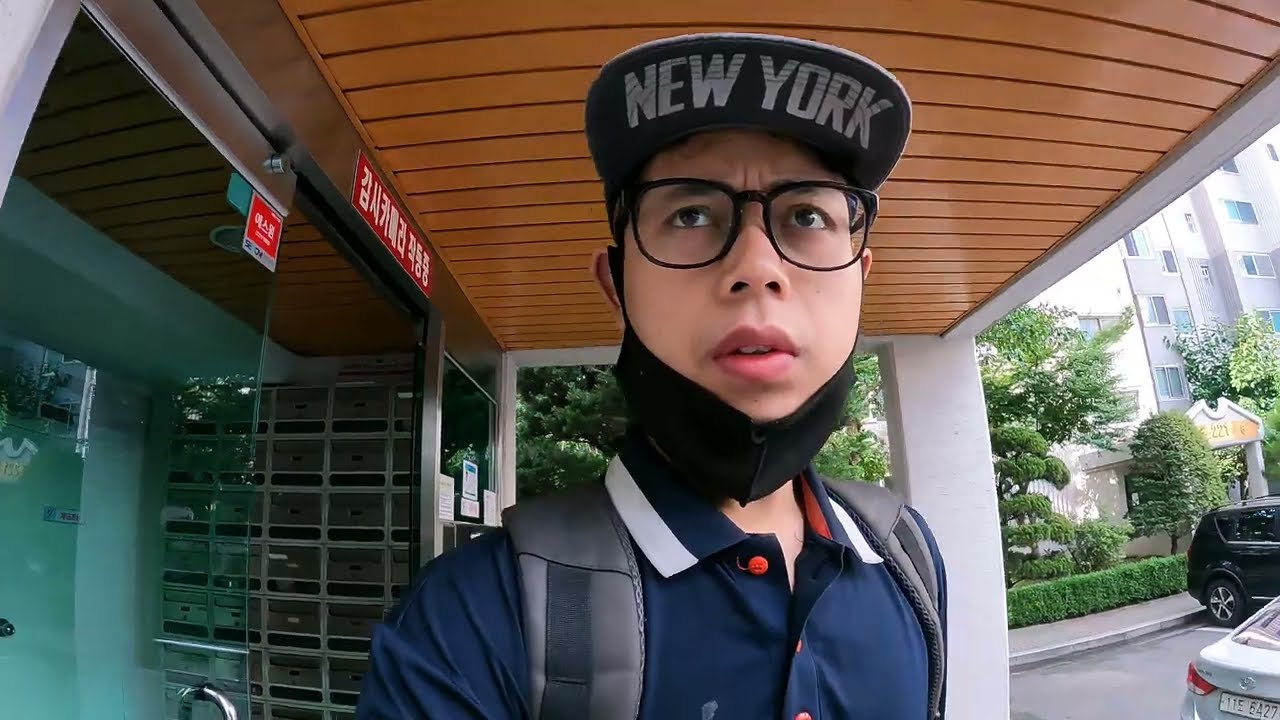The image shows a selfie of a man, possibly Hispanic, positioned from the shoulders up. He is wearing dark-framed, clear-lensed glasses and a baseball cap with "New York" inscribed on the underside of the bill. His dark eyes and eyebrows are clearly visible, and he has a black face mask pulled down to his chin. The man also sports a blue collared shirt with a white band around the collar and a red button, along with visible backpack straps over his shoulders. He appears to be outdoors, with his head turned slightly to the left.

In the background, there is an architectural setting featuring a building entrance with an overhang that looks like it belongs to either an apartment building or a hotel, indicated by a wooden-looking roof. To his left, there is a red sign with Korean script above a metal door frame, suggesting he might be in Korea. Additional background details include well-maintained shrubs, part of a black SUV, another car, and a distant building. The scene appears to be well-lit, typical of a sunny day.